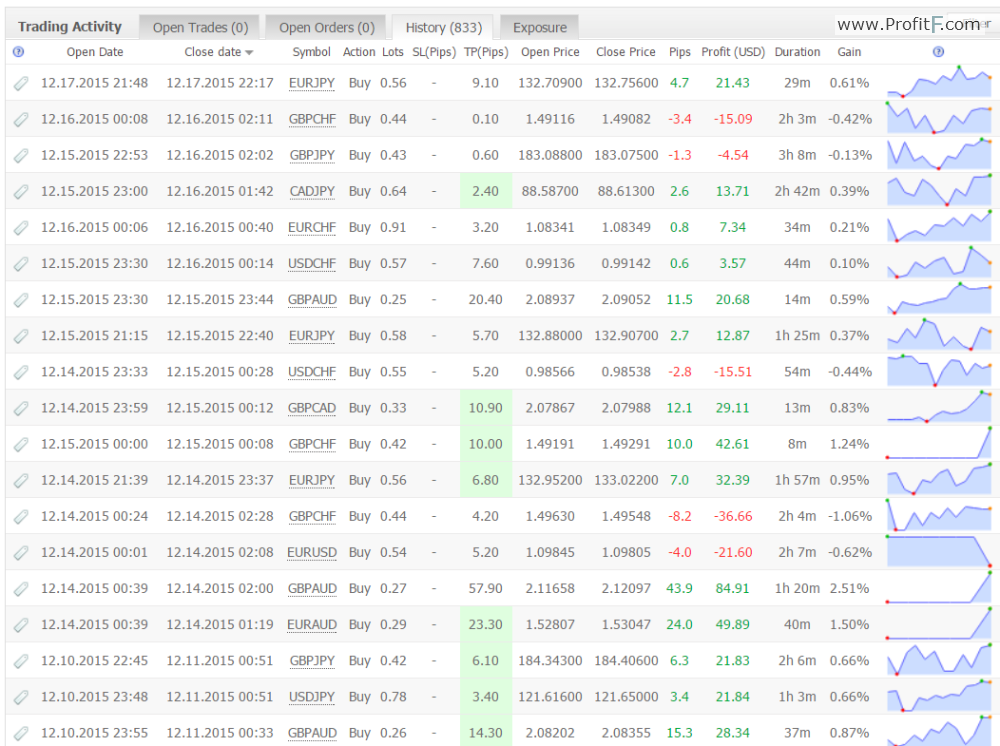A detailed image caption for the described voice input could be:

---

The image depicts a comprehensive trading interface, likely part of a stock market or forex platform, filled with extensive information. On the right side, there are numerous indicators illustrating stock performance, highlighted with red dots to mark high and low points. The interface appears to belong to someone working within a stock exchange environment engaged in active trading.

Several tabs are visible at the top, with the current tab labeled "Trading Activity." This tab presents details such as opening and closing dates and times for various trades. For instance, the first trade listed began on December 17, 2015, at 21:48, with the currency pair "EUR/JPY." It indicates a "Buy" action with the initial trade volume marked as 0.56 lot size.

The screen showcases approximately 25 entries, each with symbols, trade actions, and various numerical data points. The statistical columns provide detailed metrics, including opening prices, closing prices, pips gained or lost, profits in U.S. dollars, trade durations, and percentage gains.

A notable example is an entry with an opening price of 132.070900, a closing price of 132.75, yielding a pip gain of 4.7 and a profit of $21.43 over a 29-minute duration, resulting in a 0.61% gain. A line graph tracing price movements further visualizes each trade's trajectory from its inception to its conclusion.

Additional tabs include "Open Trades," "Open Orders," "History," and "Exposure," providing further avenues for trade management and analysis. The website address displayed at the top right corner is "profitf.com," indicating the platform's domain.

---

This detailed caption covers the critical components of the trading interface and its functionalities, making it comprehensive and informative.